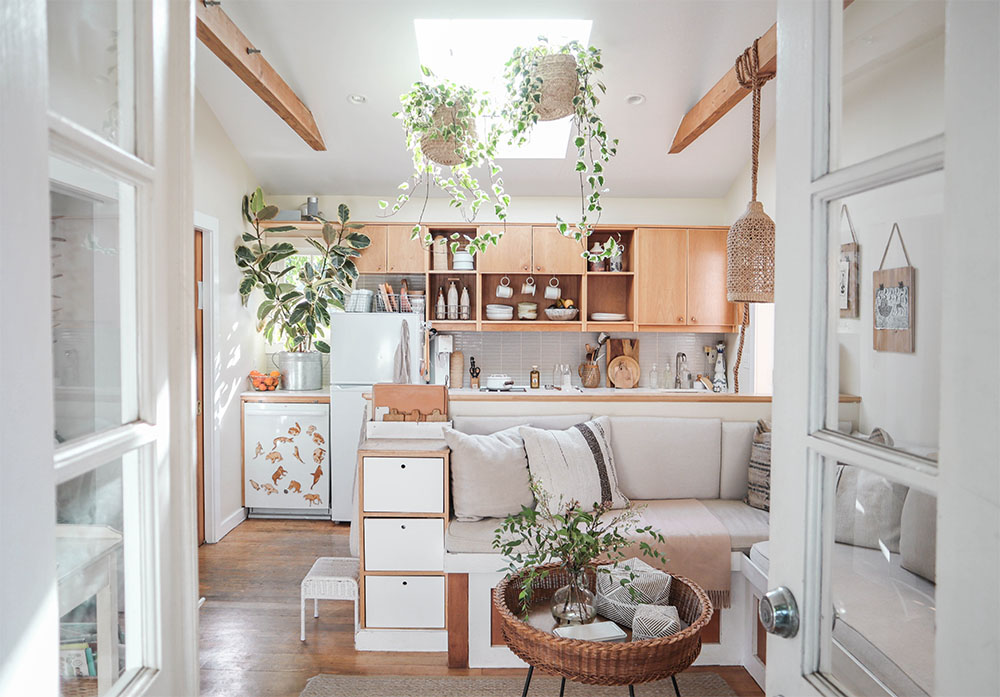This photograph captures the serene and peaceful interior of a home through a set of white French double doors. The front shows a brown basket filled with assorted items, positioned in front of a cream-colored sectional couch adorned with white pillows. The flooring is a warm, brown wood that complements the light wooden cabinetry and accent pieces throughout the space. The kitchen features wooden cabinets and white appliances, including a prominently visible white refrigerator. A rectangular skylight brightens the room with sunlit luminosity, casting a glowing light that highlights two hanging plants with trailing leaves. Additional plants are dispersed throughout, including a large one on the kitchen counter and a smaller one nestled in the basket on the floor. Wooden beams and white artwork further decorate the space, blending natural elements with a tranquil, cohesive color scheme.